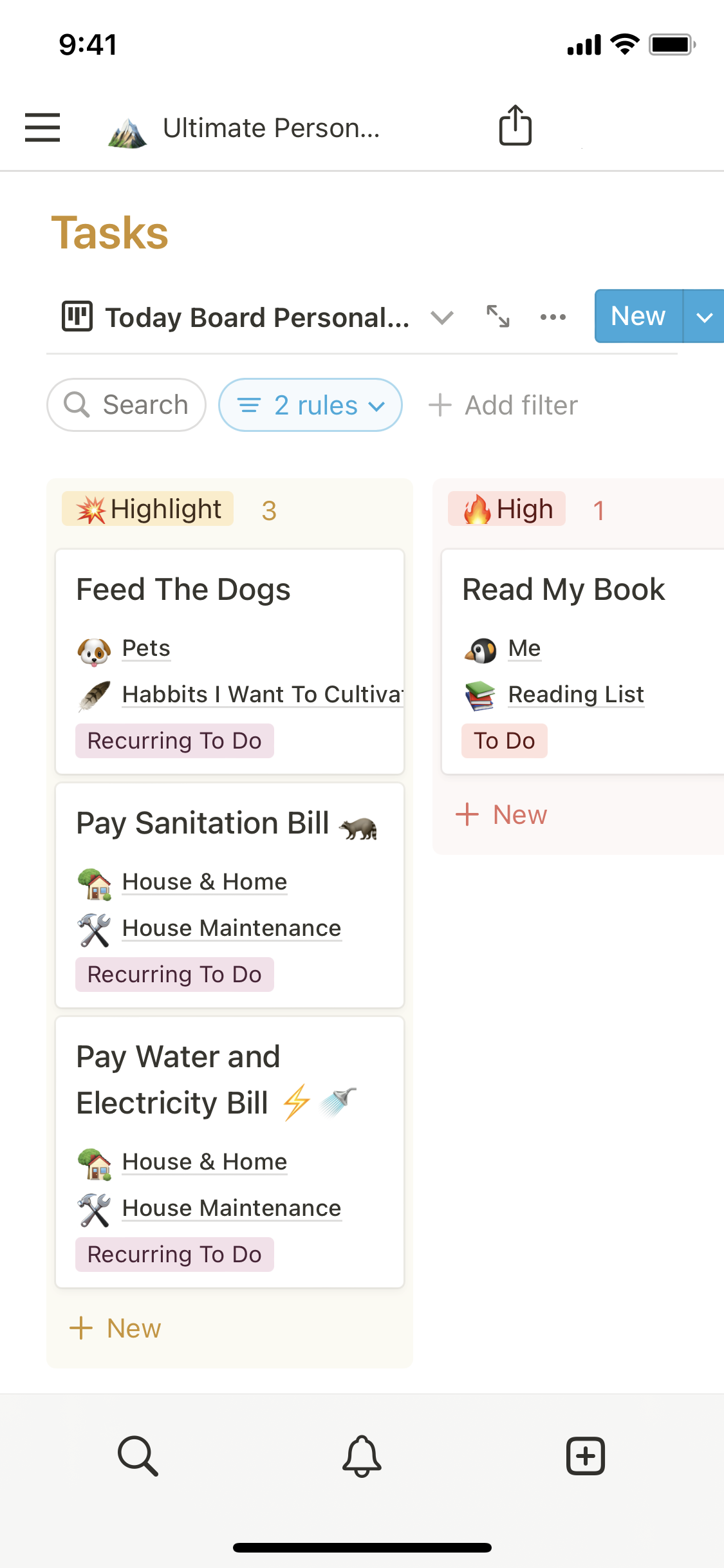This is an image of a screenshot from someone's task management app. At the top of the screen, the partially visible title suggests "Ultimate Personal," likely indicating the purpose of the app. Below this title, the word "Tasks" is prominently displayed, and underneath it is a subtitle reading "Today Board - Personal." The app interface includes filter and search icons for navigation.

The main section features four task squares, each organizing different tasks. The first task is tagged with "Highlight" and titled "Feed the dogs." Additional details describe it as part of "Pets habits I want to cultivate" and it holds a tag labeled "Recurring To-Do."

The next two tasks are both tagged "Recurring To-Do" and are titled "Pay sanitation bill" and "Pay water and electricity bill," respectively. These tasks include icons for house maintenance and home-related activities.

The fourth task stands out with a "Highlight" tag marked by a flame icon, labeled "Read my book." This task is simply tagged as "To-Do," unlike the previous recurring tasks.

This detailed organizational layout helps the user manage their daily responsibilities effectively.